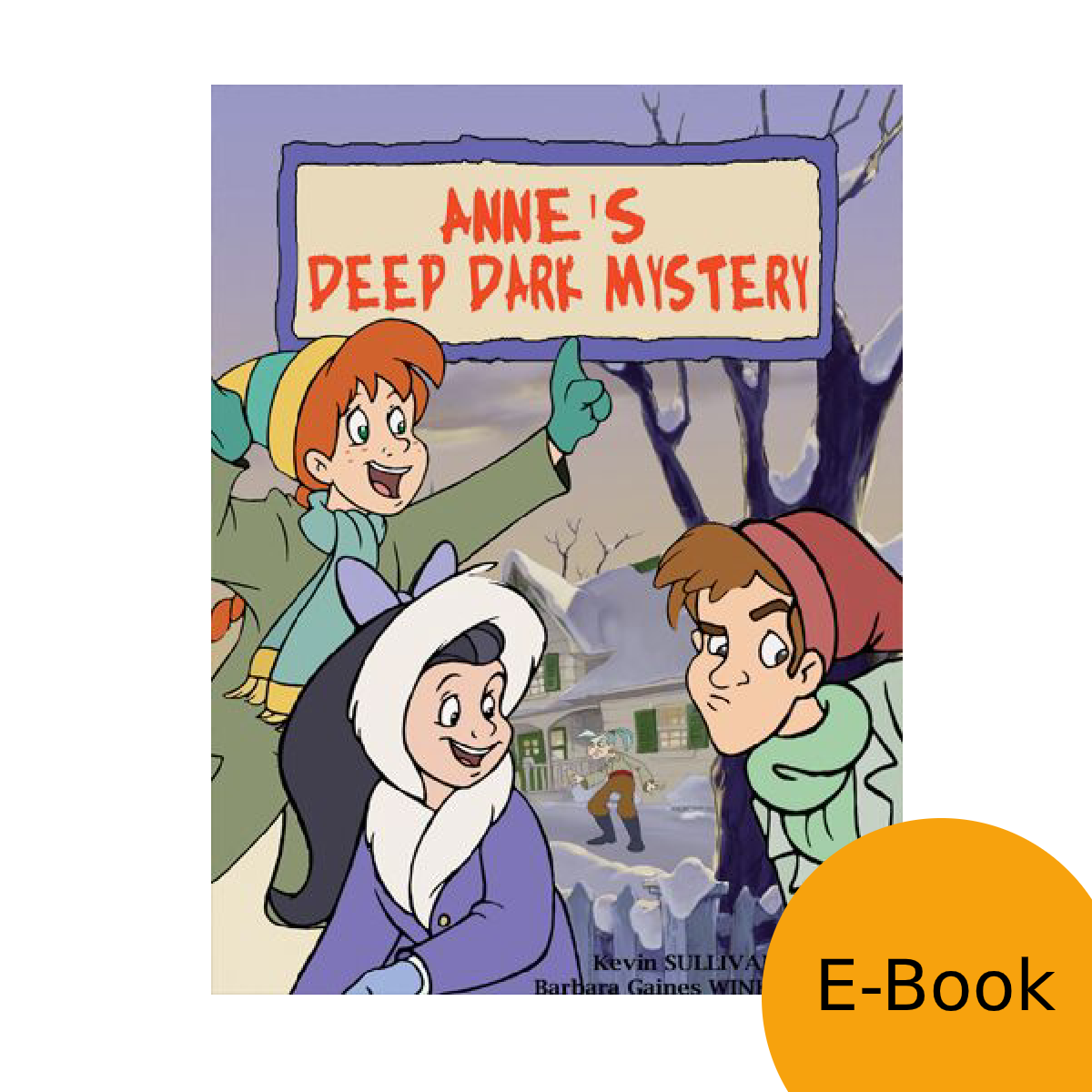The image is the cover of an e-book featuring Disney-style illustrations. Dominating the background is a large, majestic tree that towers above a charming house. In front of the house stands a man dressed in brown trousers and Wellington boots. The scene is set in a snowy landscape, adding a whimsical touch to the setting. 

In the foreground, three children are gathered near the tree. One of the children, a black-haired girl with long hair and a hood, is pointing towards a sign that presumably displays the title of the book, "Anne's Deep Dark Mystery." The girl is wearing a blue coat, creating a striking contrast with the snowy background. 

To her side stands a brown-haired boy, adorned in a green scarf and brown hat, adding to the cozy, wintry ambiance. The third child, a ginger-haired boy, is dressed in a yellow and green turquoise hat, complemented by a turquoise scarf with yellow edges and a khaki-colored coat. His look is completed with a single green glove. The scene is lively and inviting, capturing the curious and adventurous spirit of the story within.